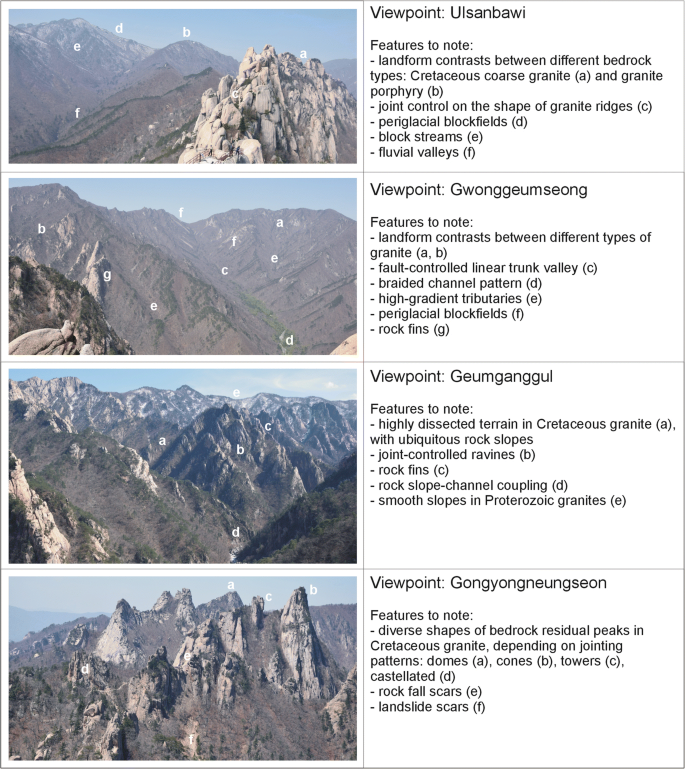The diagram, likely from a presentation or slide, depicts four distinct viewpoints of mountainous landscapes. Each viewpoint is represented by a photograph arranged in a column on the left side, labeled with white letters from A to G. The corresponding descriptions are detailed on the right side. 

1. **Viewpoint Ulsanbawi**: Highlights the landform contrasts between different bedrock types, including Cretaceous coarse granite and granite porphyry. Special note is made of the joint control on the shape of the granite ridges, the presence of paraglacial block fields, block streams, and fluvial valleys.
2. **Viewpoint Gwangwungseong**: Notes also the contrast between granite types and includes features such as a fault-controlled linear trunk valley, a braided channel pattern, high-gradient tributaries, paraglacial block fields, and rock fins.
3. **Viewpoint Gwanggangol**: Describes a highly dissected terrain in Cretaceous granite characterized by ubiquitous rock slopes, joint-controlled ravines, rock fins, rock slope-channel couplings, and smoother slopes in the Proterozoic granite.
4. **Viewpoint Gwangyongnyeongseong**: Features diverse shapes in bedrock, including residual peaks in Cretaceous granite influenced by joining patterns, as well as domes, cones, towers, castellated rockfall scars, and landslide scars.

Each viewpoint description details notable geological and geomorphological features, providing a comprehensive overview of the landscape characteristics.